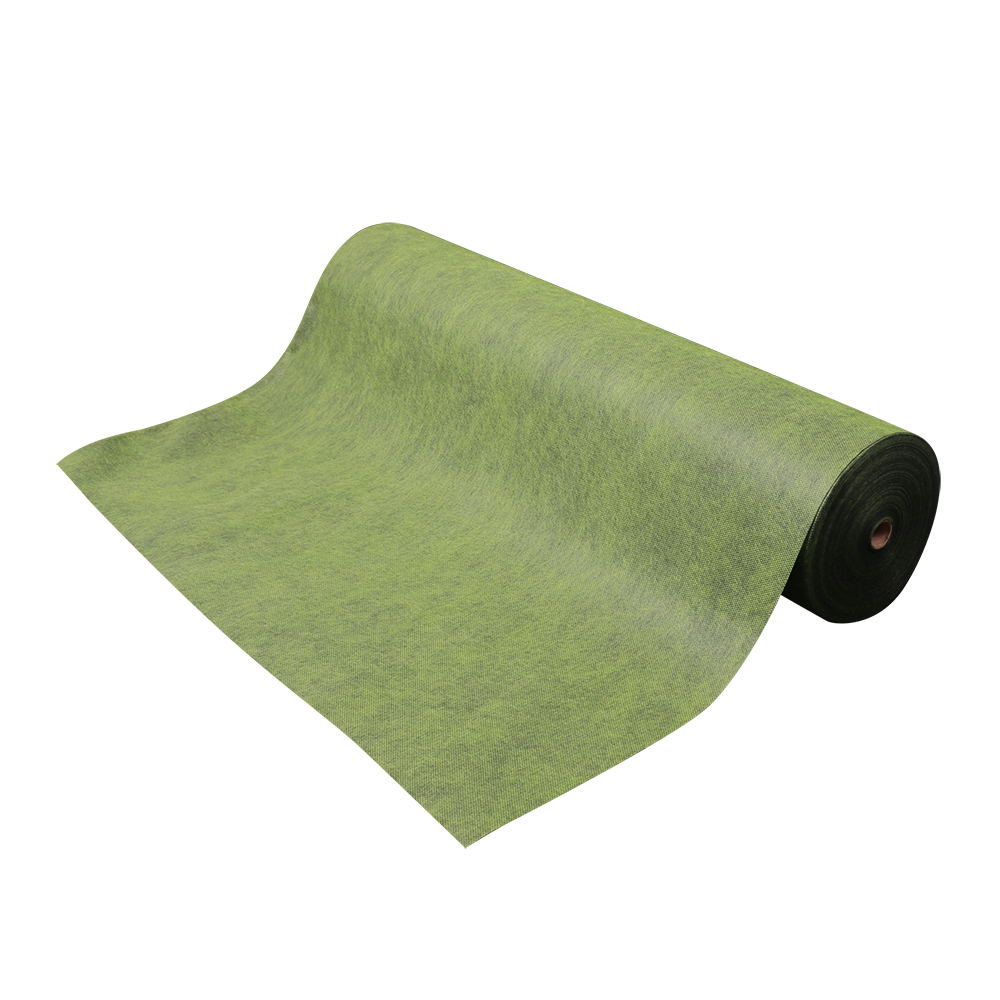This image captures a thick, angled roll of green fabric, suspended against a pure white background, giving it a clipart-like appearance. The fabric, which resembles a corduroy texture, is wrapped around a small cardboard tube at its center and is slightly unfurled with some material laid out on the surface to the left. The green hue is varied with different shades ranging from mossy greens to darker tones, reminiscent of turf on a football field, giving it a naturalistic look. The roll appears quite substantial in size, possibly encompassing a foot-long radius, and the photorealistic style offers a detailed, textured view of the fabric.